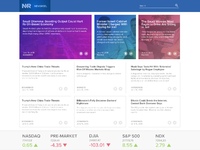This screenshot contains various visual elements organized in a structured format. At the very top of the image, there is a dark blue gradient bar featuring the initials "NR." Directly below this dark blue bar, there are three distinct rectangles. The first rectangle is purple with white text, the second is blue with white text, and the third is red with white text. Each of these rectangles displays a gradient overlay that partially reveals an underlying image.

Below these colored rectangles, there are six white squares, each containing blue text. These squares provide information related to the NASDAQ market, including specific numbers. Some of these numbers are highlighted in green with upward-pointing arrows, indicating positive changes, while others are in red with downward-pointing arrows, indicating negative changes.